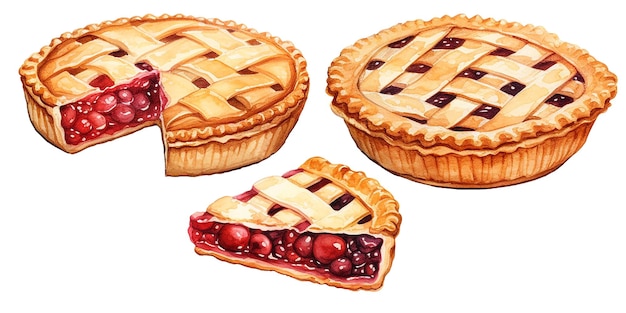This image depicts two deep-dish cherry pies with intricate lattice tops, set against a clean white background. Both pies showcase beautifully browned crusts with crimped edges, rendering a mix of tan and golden brown hues. On the right, a whole pie with a golden brown lattice crust reveals glimpses of its rich, red cherry filling beneath the woven strips. To the left, another pie has a triangular slice cut out, exposing a luscious interior filled with cherries in a syrupy sauce. This cut piece is prominently displayed in the forefront, demonstrating the detailed lattice top and vibrant cherry filling. The pies appear slightly stylized, blending realistic elements with a cartoon-like design.